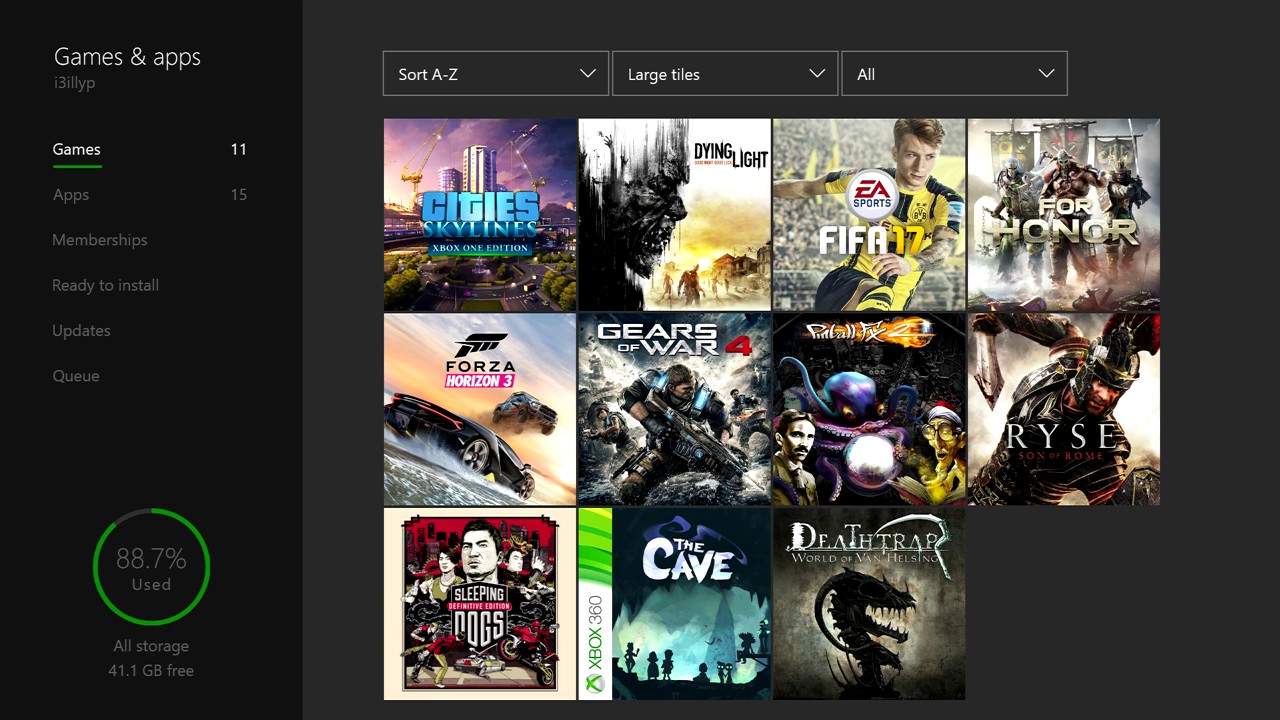The image captures a screenshot of a black-themed games and apps store interface. In the upper left-hand corner, white text reads "Games & apps." The user's profile under the name "i3illyp" is visible. 

The interface is divided into several menu categories: "Games," "Apps," "Memberships," "Ready to install," "Updates," and "Queue." The "Games" category is currently selected, indicated by white text, while the other categories are grayed out. To the right of "Games," the number "11" signifies that 11 games are available. Similarly, the "Apps" category, which is grayed out, shows the number "15," denoting 15 available apps.

At the bottom of the screen, a green circle displays the storage usage, showing 88.7% full. Inside the circle, the percentage "88.7%" is prominently displayed. Below this, the text "All storage" indicates that 41.1 gigabytes of storage space is free.

To the right of the interface, there are thumbnails of various games organized in three rows. The first and second rows each contain four game thumbnails, while the third row at the bottom has three game thumbnails.